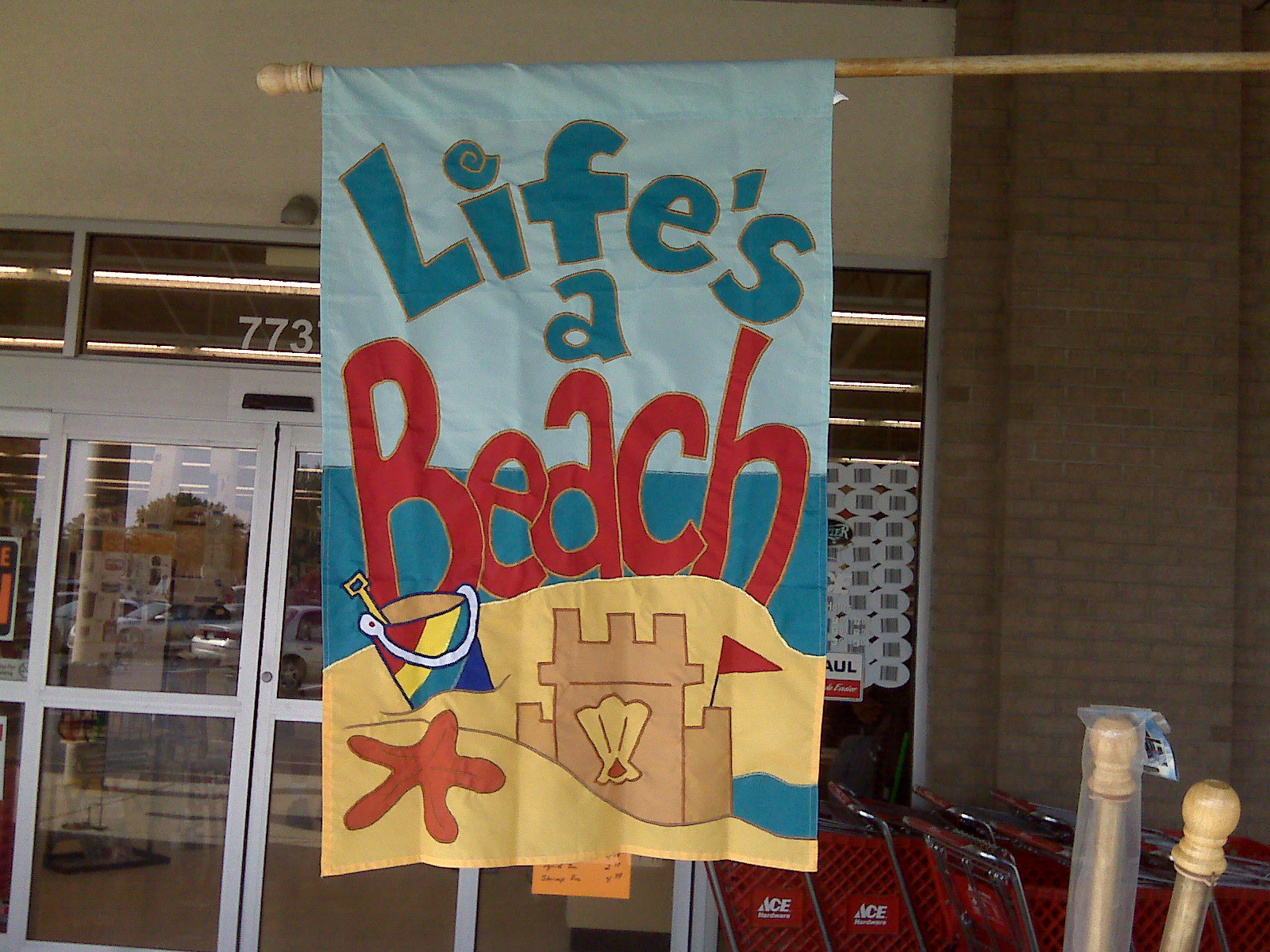The photograph captures a vibrant flag displayed on a wooden rod, extending from the right side of the frame. The flag vividly declares "Life's a Beach" with the words "Life" and "A" in blue, and "Beach" in red, all constructed from patchwork fabric. The scene depicted on the flag showcases a sandy yellow beach adorned with a detailed brown sandcastle, topped with a decorative shell and a red flag. An orange starfish and a multicolored bucket, featuring red, yellow, green, and blue hues with a white handle and a yellow scoop, enhance the playful seaside imagery. In the background, dark blue water meets the light blue sky. 

Behind the flag, the setting transitions to the front of a supermarket, identified by its glass sliding doors and the number 773 prominently displayed in white on the windows. To the right, a brick wall and a lineup of red shopping carts with silver accents are visible, further confirming the commercial location.